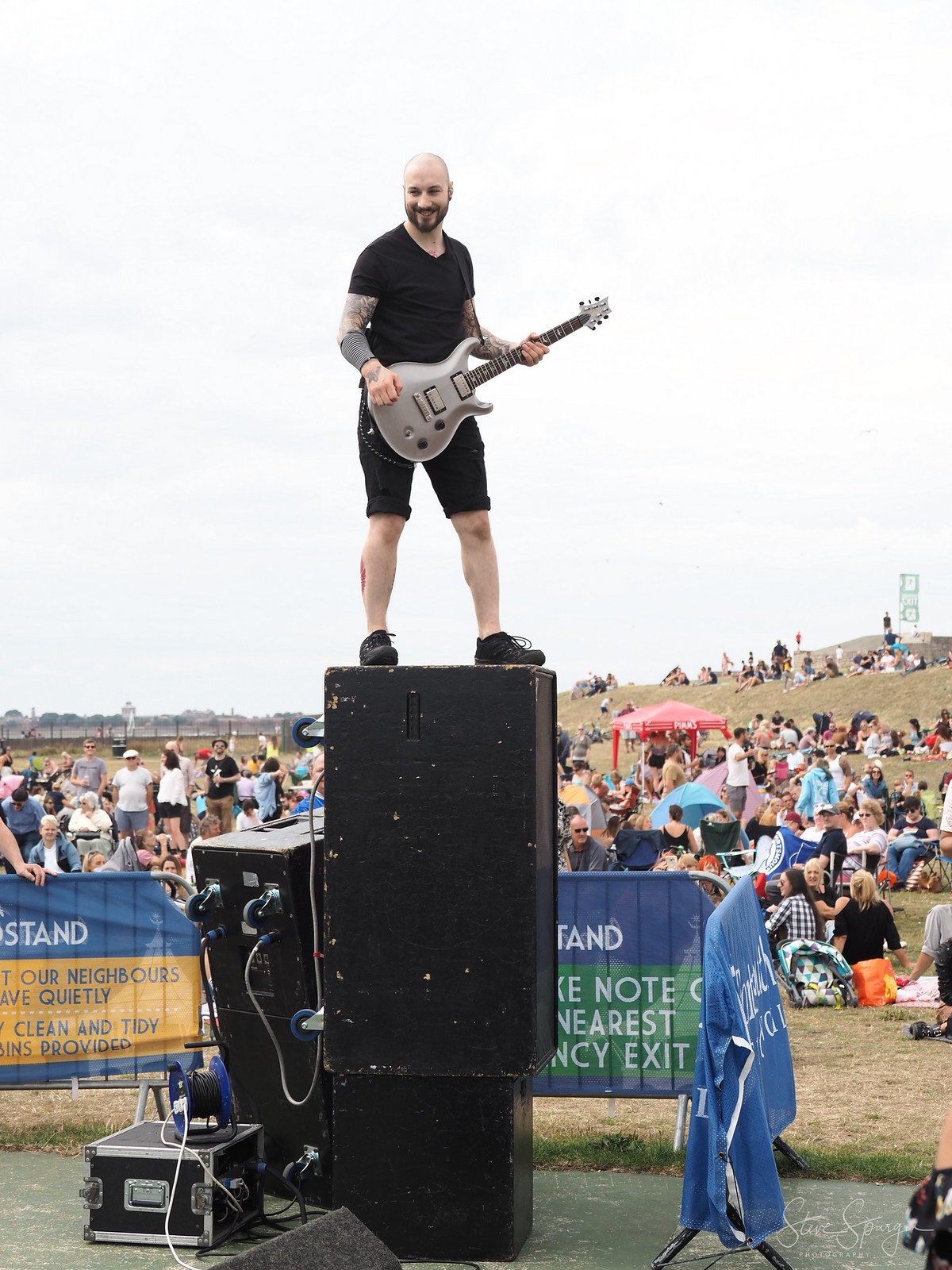The photograph captures a musician, bald with a beard, standing atop a large amplifier that is stacked on another amplifier. He is performing at an outdoor concert, holding an electric guitar and smiling. Dressed in a black t-shirt, black shorts, and black sneakers, he stands elevated above an audience. The crowd is spread across rolling hills with some individuals seated on lawn chairs or directly on the ground, among umbrellas and patches of brownish sand. Signage around the venue includes partially visible text mentioning phrases like "stand," "our neighbors," "quietly," "clean and tidy," and "emergency exit." Additional speaker boxes with tangled wires are situated next to the main amplifier setup, contributing to the casual and lively outdoor concert ambiance.